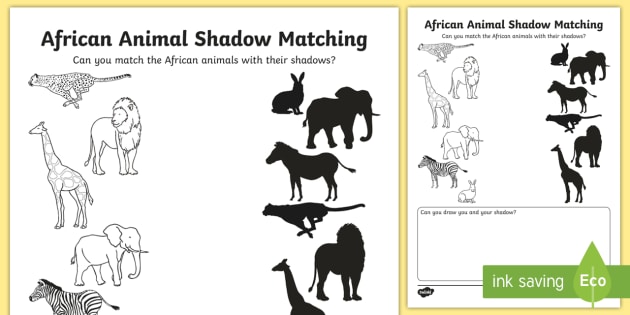The image depicts an educational activity page titled "African Animal Shadow Matching," designed for children. The main task is to match the outlined drawings of various African animals—such as a cheetah, lion, giraffe, elephant, and zebra—with their corresponding blacked-out silhouettes on the right side. The activity page is mostly in black and white and includes two different perspectives of the same content: a full-page view and a smaller, eco-friendly version labeled with an "Ink Saving Eco" stamp, indicating it can be printed with minimal ink usage. The instructions prompt the child to match the outlines with the shadows, followed by an additional task that asks, "Can you draw you and your shadow?" This interactive sheet appears to be both an educational tool and a fun activity, likely intended for classwork or homework assignments to engage children in learning about African wildlife.